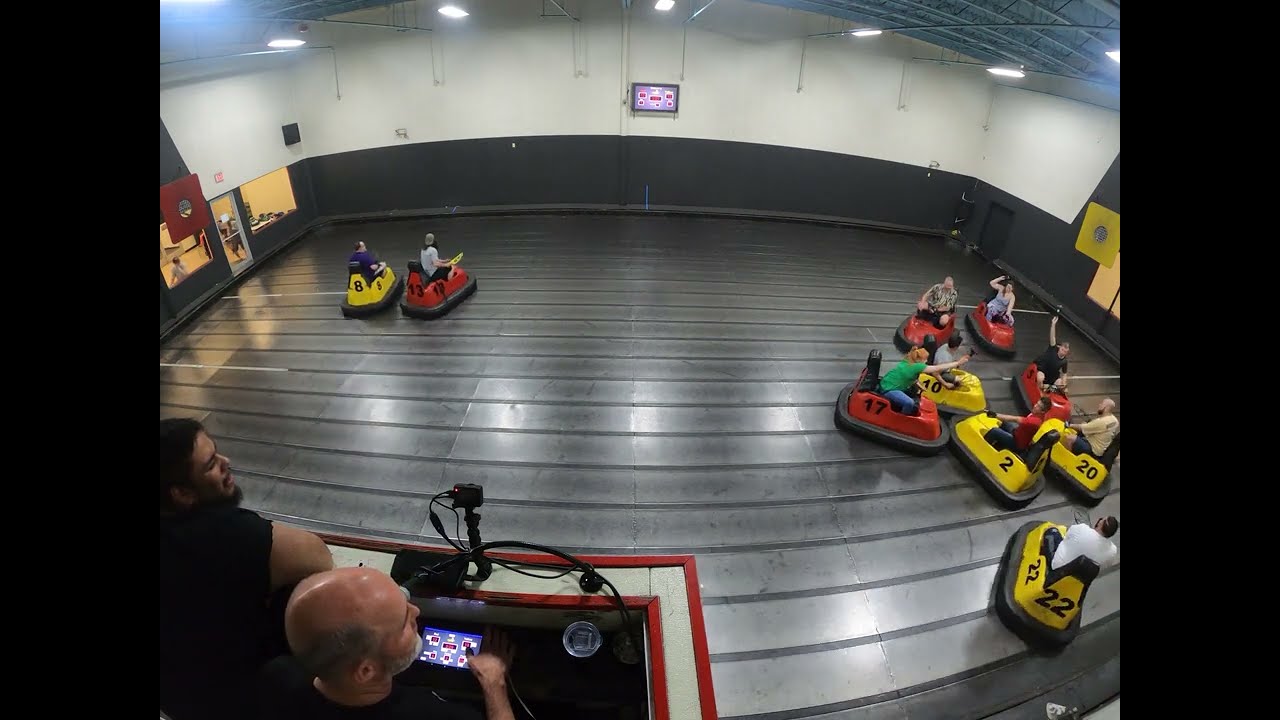The image depicts an indoor bumper cars arena with a high vantage point that looks down on the action. The area, housed in a room with an unfinished metal-beamed ceiling, features a gray and black striped floor. The bumper cars, some red and some yellow, are numbered—visible numbers include 2, 8, 10, 13, 17, 20, and 22. A cluster of around ten adults, likely between their 30s and 50s, are seen driving and colliding in their cars predominantly on the right side of the arena, creating a chaotic pile-up. In contrast, a pair of bumper cars—a red one and a yellow one—are leisurely navigating on the left side. 

In the bottom left corner of the image, a small control booth is visible where two operators are stationed. One is a bald white man, while the other man, wearing a black t-shirt, has black hair and a beard. This booth seems to have technological equipment, including a GoPro setup and possibly an iPad, indicating they might be recording the activity or controlling the ride. The walls of the arena are white with a black trim at the bottom, adding to the structured yet playful environment of the indoor amusement center.